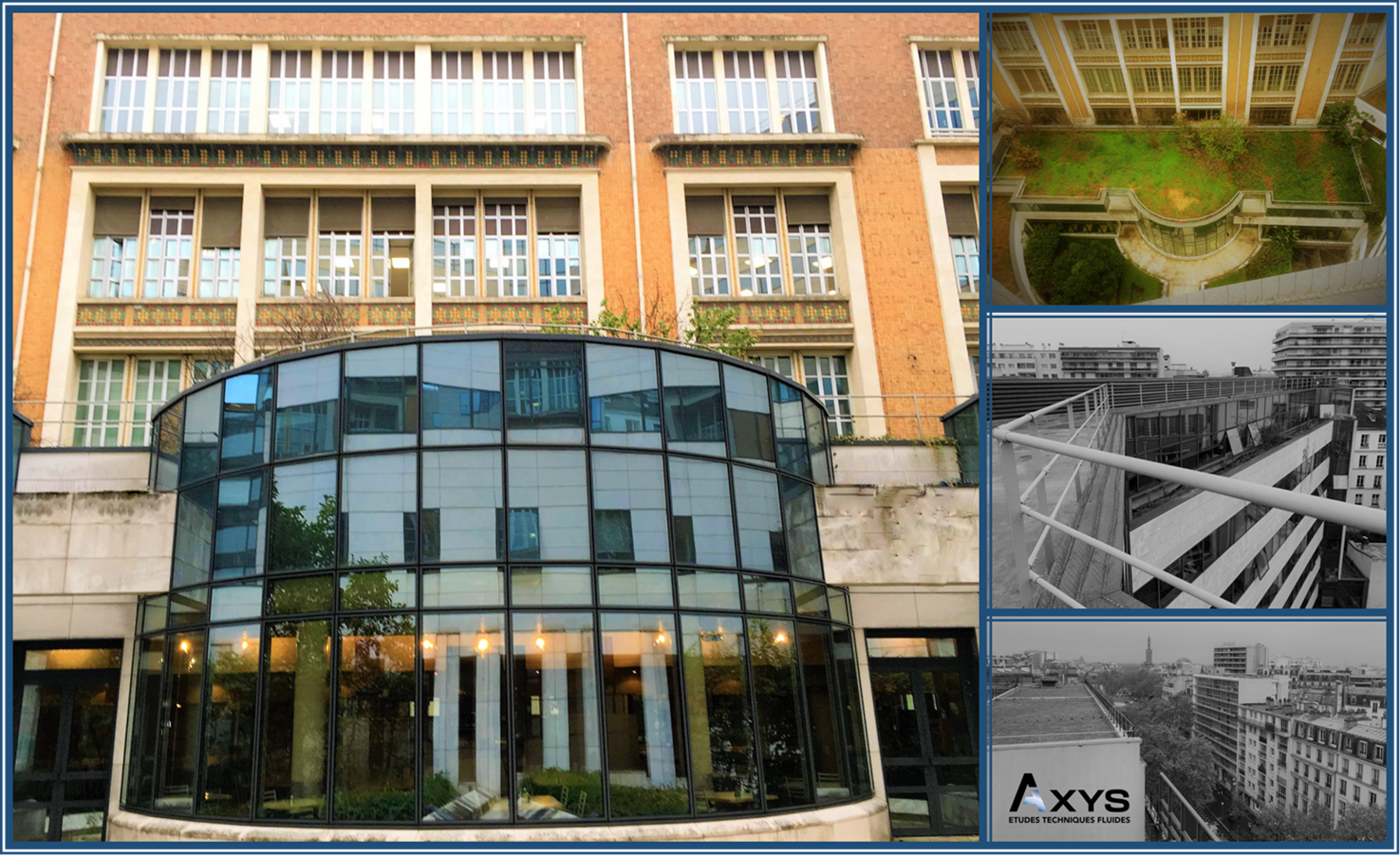This composite image displays an extensive collage focused on a particular building and its surroundings. The largest image dominating the entire left side features a four-story red brick edifice with numerous white-framed windows. This structure is accentuated by a half-glass dome that covers its entrance, adding a modern touch to the otherwise classic architecture. Adjacent to this, in the top right corner, an aerial shot gives an overhead perspective of the same building, revealing a lush courtyard adorned with grass and small plants. Below this aerial view are two black-and-white photographs capturing additional buildings, possibly historical images of the same or related structures. The bottommost photograph includes text that reads "A-X-Y-S, Studies, Technique, Blitz." The collage is imbued with diverse colors such as brown, white, various shades of blue, yellow, black, gray, green, and orange, creating a vibrant yet historic ambiance. The well-organized layout and the blend of contemporary and historical elements suggest a meticulous and comprehensive presentation of the building and its evolution over time.